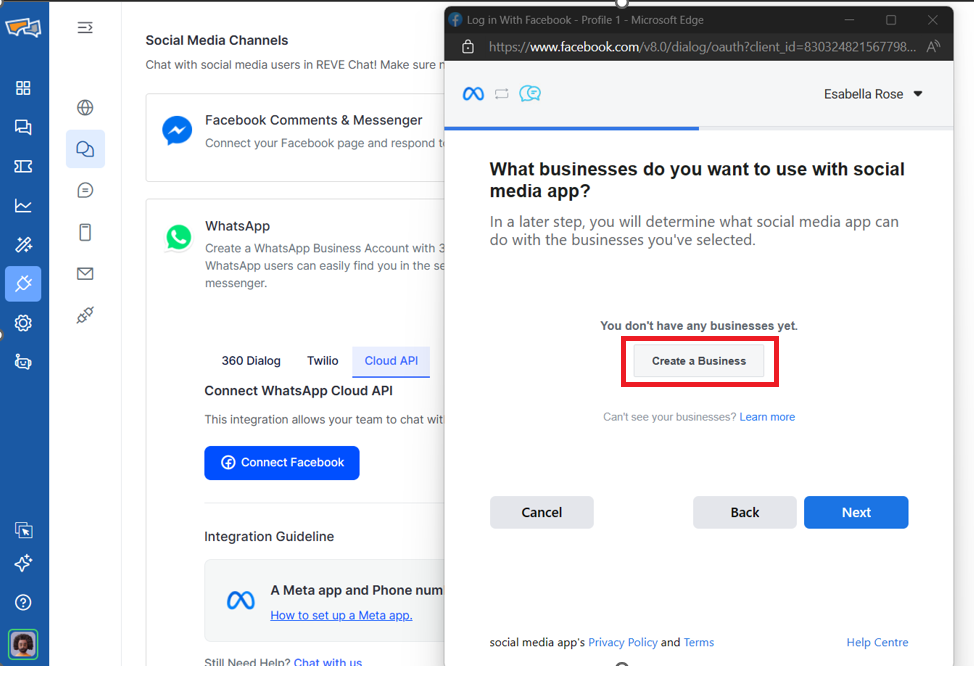The image shows a digital interface split into two sections: a computer settings page on the left side and a Facebook page overlay on the right side.

### Left Side (Computer Settings Page)
- **Header:** "Social Media Channels"
- **Content:** 
  - A section titled "Chat with social media users and you leave chat." The text following this is cut off by the Facebook overlay.
  - Another section reads, "Facebook Comments and Messenger: Connect your Facebook page and respond."
  - Below that, there is a WhatsApp icon with the text: "Create a WhatsApp business account. WhatsApp users can easily find you." The following text is partially obscured.
  - Further down, it mentions "360 dialogue," "Twilio Cloud API," and "Connect WhatsApp Cloud API."
  - A conspicuous blue button labeled "Connect Facebook."
  - At the bottom, there's text reading "Integration Guideline."

### Right Side (Facebook Page Overlay)
- **Address Bar:** Displays a Facebook URL.
- **Profile Name:** "Isabella Rose" is shown at the far right.
- **Content:**
  - A prompt asking, "What businesses do you want to use with the social media app? In a later step, you will determine what the social media app can do with the businesses you selected."
  - A note stating, "You don't have any businesses yet."
  - A red-bordered section with loose text inside that reads, "Create a business."
  - An option labeled, "Can't see your businesses? Learn more."
  - Buttons for navigating options: "Cancel," "Back," and a highlighted "Next."

This detailed description helps in visualizing the dual interface focused on incorporating Facebook functionalities within a broader social media management system.